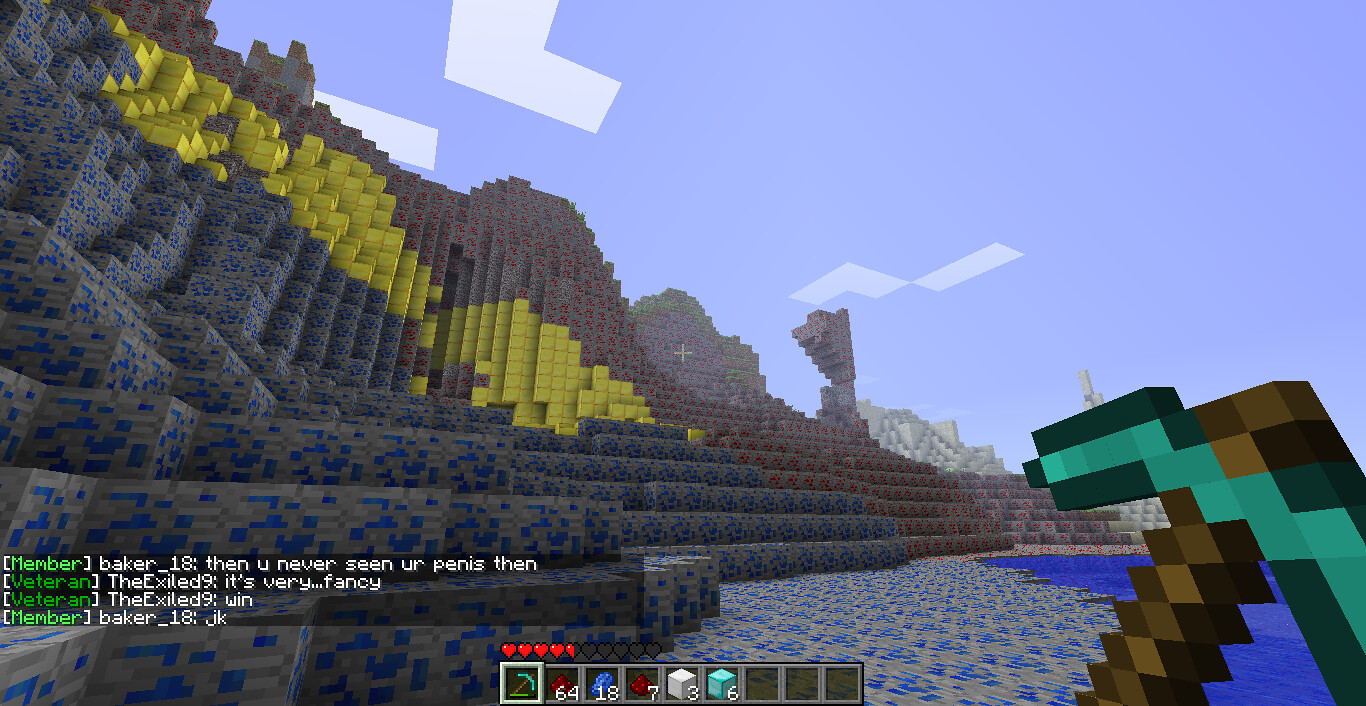This is a highly pixelated screenshot from a video game. A brown weapon with light and dark teal accents extends from the bottom right corner of the screen. Along the bottom middle, a bar displays numbered squares containing various objects. Above this bar, there is an indicator showing four and a half red stars or hearts. On the right side of the screen, pixelated water can be seen, while the left features steps leading up a hill. The text in green at the bottom left reads "member, veteran, veteran, member, baker." Below this, it states "veteran is exiled," followed by "exiled" and "baker" once more.